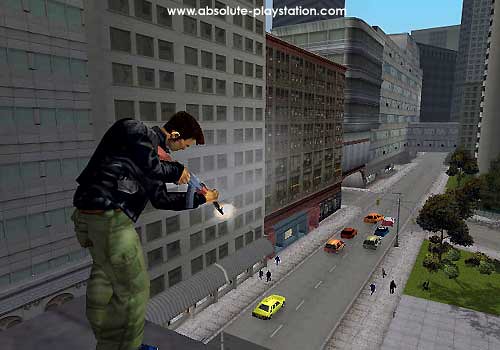The image is a high-quality screenshot from a video game, displaying a detailed urban scene. At the top of the image, the URL "www.absoluteplaystation.com" is prominently shown. The image, which is about 20% wider than it is tall and slightly compressed with some background artifacts, features a man standing on a gray ledge near the upper left corner. The man, who is facing away at an angle between one to two o'clock, is dressed in a black leather jacket, green camouflage pants, and a tactical vest. He holds an automatic rifle emitting a bright muzzle flash, indicating he is in the act of shooting. The street below him extends towards the back of the image and is lined with gray commercial buildings on the left. The road is populated with several cars in bright colors, including yellow, red, and orange, and flanked by grassy areas interspersed with trees and parks on the right. The sidewalks on either side feature small dots representing people, with six visible at different distances. The urban backdrop completes the setting with a mix of office buildings and skyscrapers, suggesting a busy city environment.